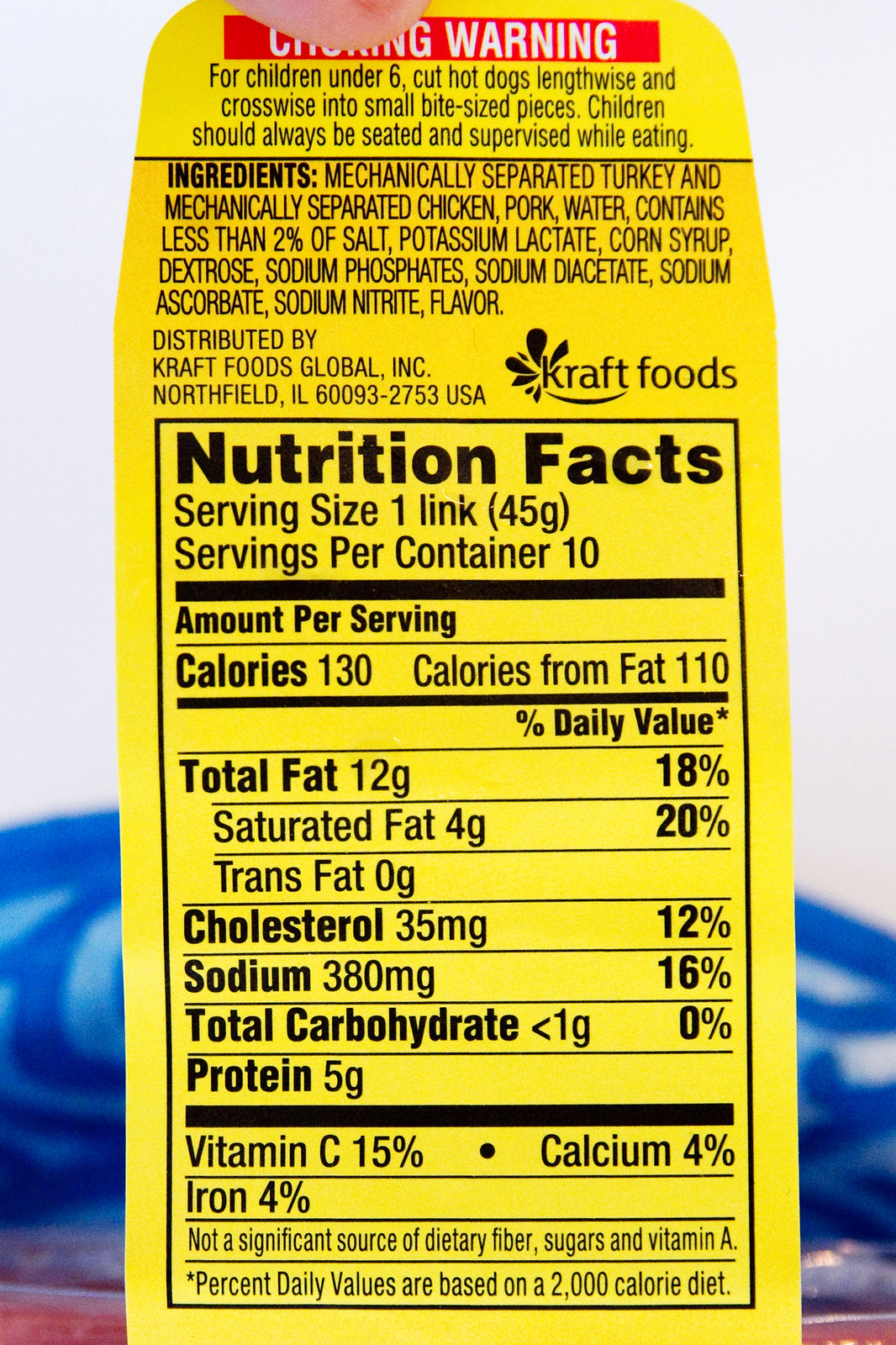This vivid, color photograph prominently features a bright yellow Nutrition Facts label typically found on hot dog packaging, possibly from a brand like Oscar Mayer. Oriented vertically, the label captures the viewer's attention against a blurred background and is accentuated by a swirling blue, white, purple, and pink design at the bottom. The top of the label displays a red warning strip cautioning about choking hazards for children under six, advising to cut hot dogs lengthwise and crosswise into small bite-sized pieces. Below the warning, the ingredients list is provided, noting mechanically separated turkey and chicken, along with various additives such as potassium lactate and sodium phosphate. The label is associated with Kraft Foods. Most of the label's real estate is taken up by a black-bordered box detailing the nutritional information, including calories, total fat, cholesterol, sodium, total carbohydrates, and protein, along with specific percentages for vitamin C, calcium, and iron.